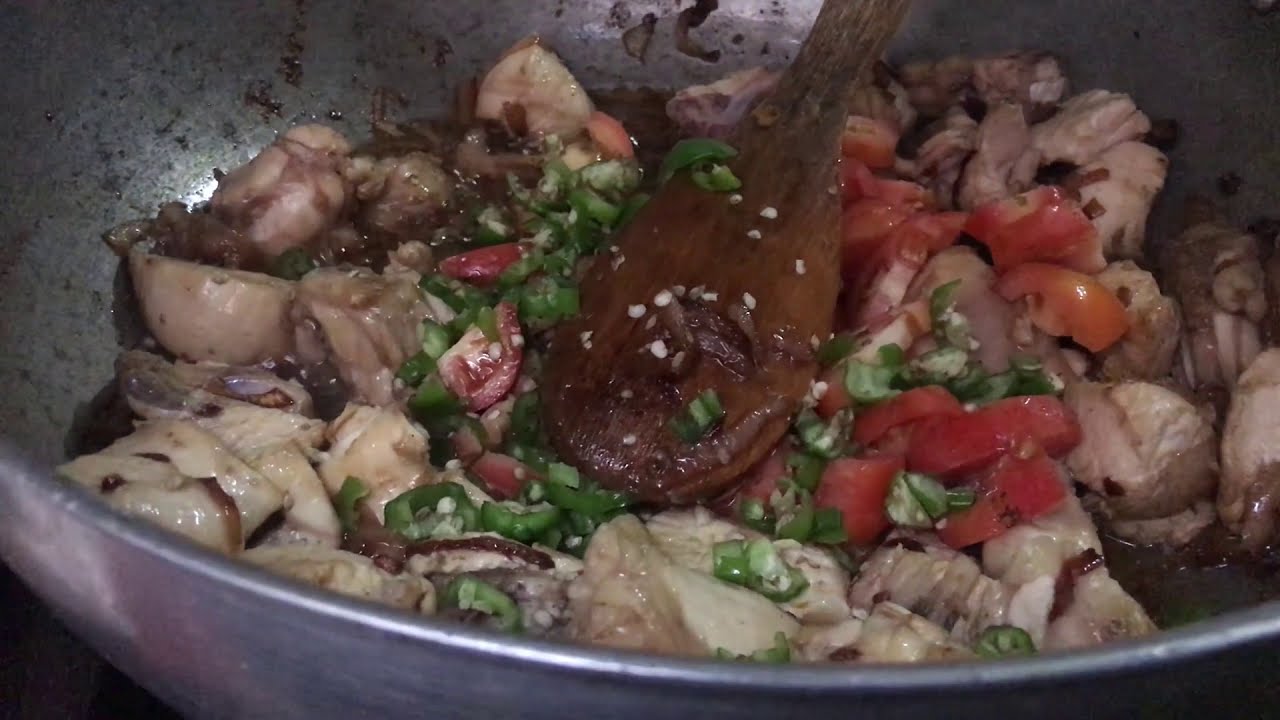A close-up image of a metal skillet reveals a vibrant dish featuring a mix of diced tomatoes and green peppers, prominently displayed on top. Pieces of chicken are scattered throughout, complemented by white onions visibly interspersed. A wooden spoon, resting across the skillet, bears remnants of the mixture, including seeds from the chopped peppers, indicating it has been actively used for stirring. The dish appears nearly cooked, with the chicken showing signs of readiness.